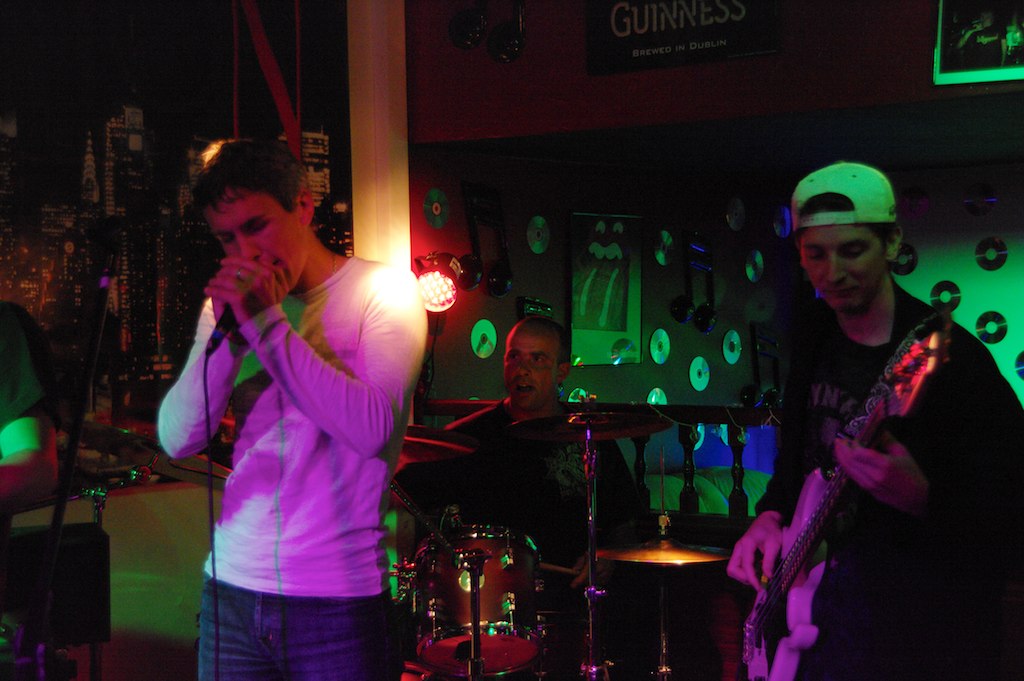The image captures a lively musical performance, likely set in a dimly lit club adorned with a variety of decorations. On the left side stands a male singer, clad in a white t-shirt and jeans, gripping a microphone with both hands, singing passionately. Beside him is a half-visible hand extending from the left edge of the frame, suggestive of another performer. Centrally placed is the drummer, energetically poised with drumsticks in hand, sitting next to a drum set. To the right, the guitarist, distinguished by his white baseball hat worn backwards and dark t-shirt, plays a white guitar. The background features a wall decorated with numerous CDs taped to it and a sign reading "Guinness brewed in Dublin", contributing to the club's vibrant ambiance. Additionally, a section of the wall is illuminated with green light, showcasing various artifacts and cityscape imagery, further enhancing the scene's eclectic feel.